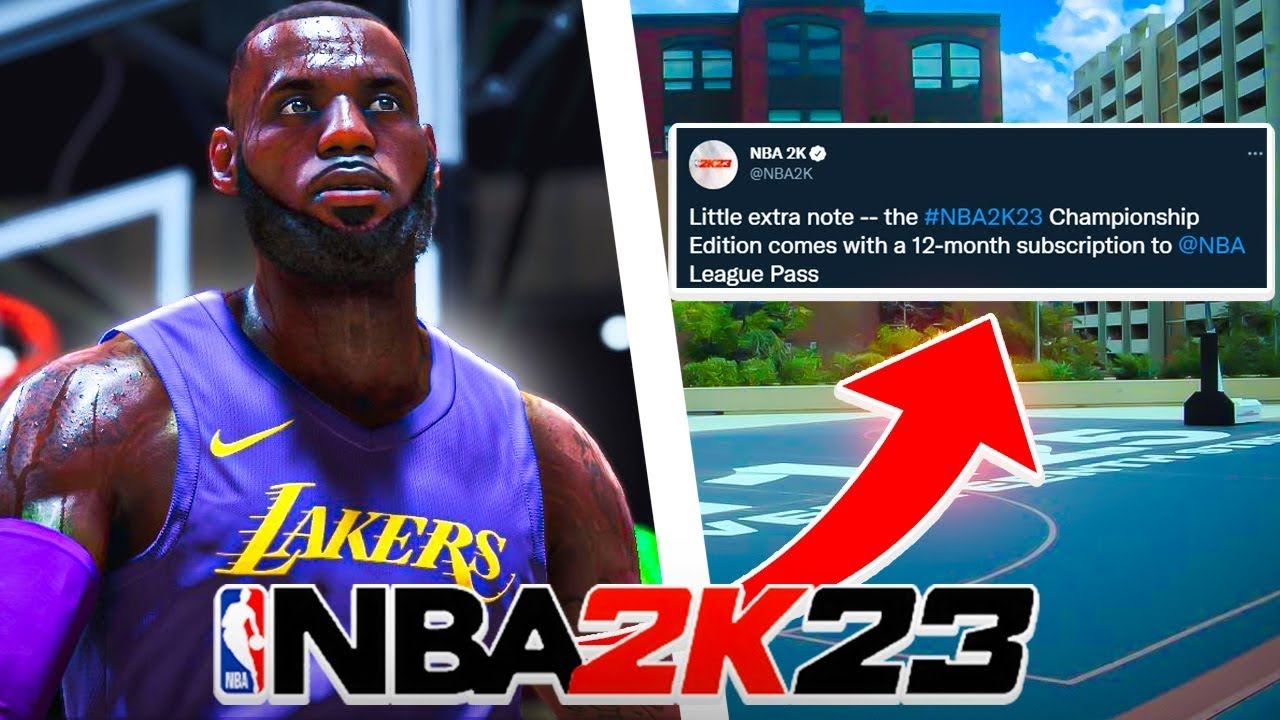In the foreground, a professional basketball player from the Los Angeles Lakers is prominently displayed. He is an African American athlete, wearing the team’s classic purple tank top adorned with a yellow Nike swoosh and the word "Lakers" emblazoned across the chest in yellow. His skin is dark and shiny with sweat, and he has short, black hair. The player sports a beard and a slight mustache, although it is difficult to ascertain whether he is wearing a mask over his chin. He also wears a purple shoulder or upper arm brace.

At the bottom of the image, the text "NBA2K23" is prominently featured. "NBA" is in black and outlined in white, "2K" is in red and outlined in white, and "23" is in black outlined in white. A significant red arrow, outlined in white, points upwards. To the left of the "N" in "NBA," the recognizable NBA logo appears, showcasing a white silhouette of a basketball player against a blue and red background, also outlined in white.

An additional caption reads: "NBA 2K23 Championship Edition comes with a 12-month subscription to NBA Elite Pass," in white letters, with "#NBA2K23" and "@NBA" highlighted in blue.

Above this, the handle "@NBA2K" is displayed alongside a verified checkmark within a white circle and the "NBA2K23" logo in red. The background depicts a stylized outdoor parking area with buildings, presented as a drawing. This detailed scene serves as a promotional image for the "NBA2K23 Championship Edition."